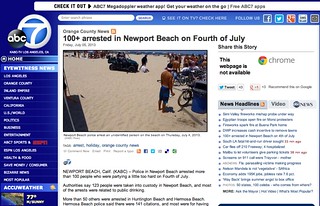This is a compact, square-shaped screenshot of the ABC7 website's front page. Dominated by a blue theme, the page features a prominent blue header and a blue sidebar on the left. The main content area on the right has a white background, enhancing readability. At the top is the headline of the featured story, accompanied by a small thumbnail image situated to the left of the headline. Below the headline is the story's text.

To the far right, there's a panel that displays the Chrome logo and a message starting with "This webpage is something," followed by social media options for tweeting or sharing the article. Below these options, a vertical list showcases additional stories from ABC, categorized both nationally and locally.

In the top left corner of the screenshot is the ABC7 logo. Directly beneath it, the label "Eyewitness News" appears, with several clickable categories listed underneath it, providing easy navigation across different sections of the website.